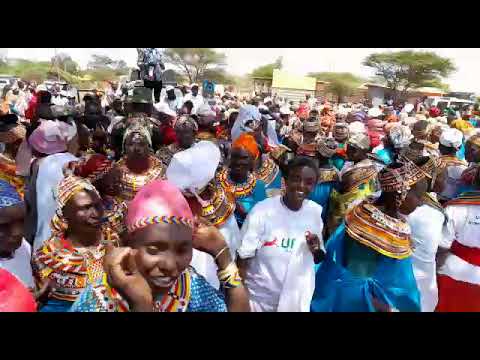This vibrant and bustling outdoor scene captures a large gathering of around 100 people, predominantly of African descent, celebrating together in an African city, possibly in Nigeria. The crowd is packed densely towards the bottom of the image, filling the space with colorful traditional garments and accessories, including head coverings, necklaces, beads, and collars that extend over the shoulders. The attendees wear a mix of traditional African clothing and contemporary attire like plain white shirts and t-shirts. The air is filled with joy and movement as many people appear to be dancing and smiling.

In the background, we can see some buildings, trees, and a statue, although the details of the statue are not clear. The sky above is mostly white, as if blotted out. The rich array of colors present in the image includes pink, blue, yellow, red, green, black, brown, and tan, making for a lively and vivid scene. The top of the image shows the sky and trees, while the lower section is dominated by the celebratory crowd. The entire scene is framed by plain black borders at the header and footer, adding a stark contrast to the colorful festivities captured in the middle of the day.